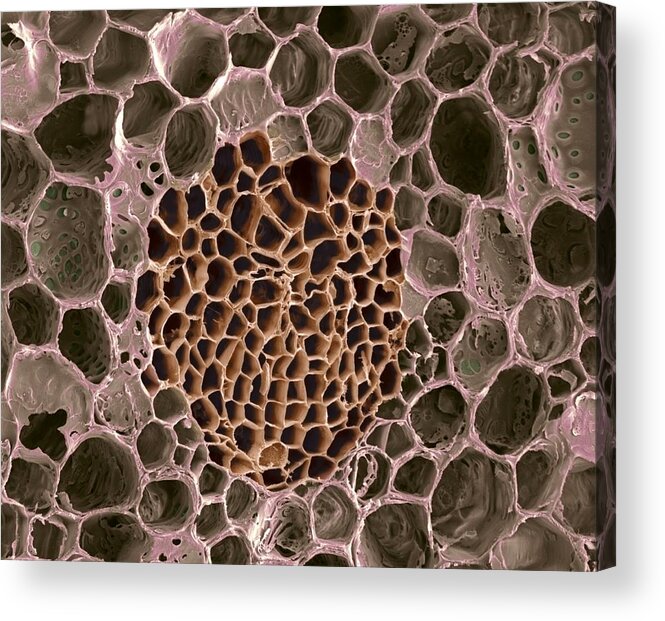The image displays a detailed close-up of a structure resembling a honeycomb, possibly from a colony of wasps or bees. At the center, tightly clustered smaller honeycomb cells in shades of light and dark brown with black interiors create a dense, textured focal point. Surrounding this central area, larger honeycomb shapes, appearing perforated with some closed-off cells, form an encircling pattern in varying hues of gray, light gray, and white. This intricate assembly of cells and tunnels, cutting through the entire frame, evokes the impression of being sliced open, revealing the internal compartments and complex organization of the colony. The overall color palette transitions from the darker, brownish tones in the middle to lighter, grayer tones on the periphery, creating a visually captivating and detailed composition that hints at the natural architecture of hive structures.